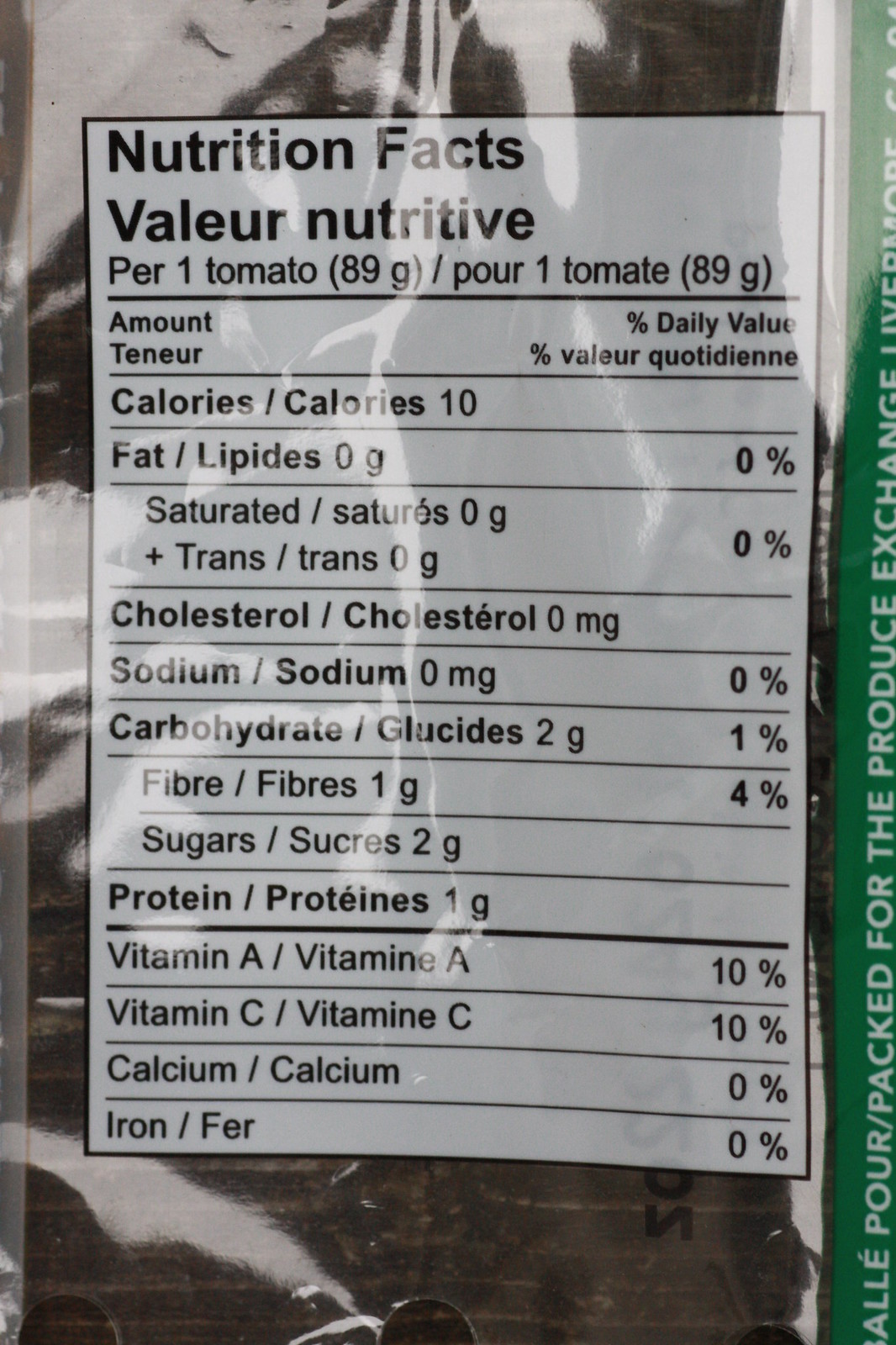This image is a close-up photograph of clear plastic food packaging that displays the Nutrition Facts in both English and French. The white label with black text indicates typical nutritional information, such as 10 calories per serving, 0 fats, no cholesterol, no sodium, 2 grams of carbohydrates (though it lists 1 gram of fiber and 2 grams of sugars, which adds up to 3 grams), and 1 gram of protein. The label specifies these values for a serving size of one tomato (89 grams), even though the actual contents inside the package appear to be bread crusts rather than tomatoes. On the right edge of the packaging, there is a green border with partially visible white lettering that includes phrases such as "Allee Poor" and "packed for the produce exchange." The layout features a clear demarcation, with the Nutrition Facts headline prominently displayed in both languages: "Nutrition Facts" in English and "Valeur Nutritive" in French. Additionally, it mentions the daily value percentages for fiber (4%), vitamin A (10%), and vitamin C (10%), with no calcium or iron.